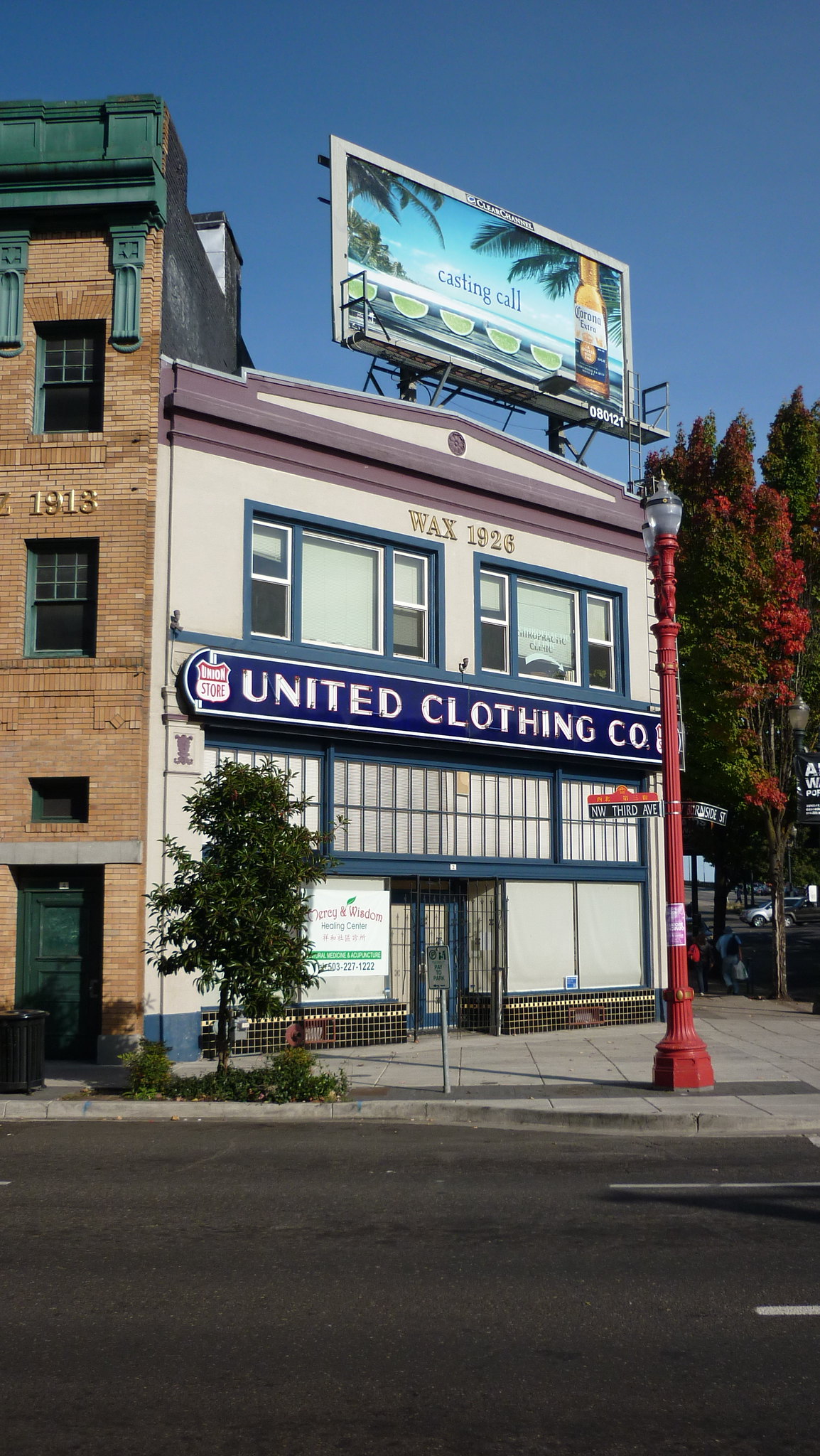This daytime photograph captures an urban street scene characterized by a white, two-story building situated at the corner of the street, angled prominently in the frame. At the bottom of the image, the street features white painted lines and appears notably empty. A sidewalk runs further up, on the right side of which stands a red-painted streetlight pole with street signage. The focal white building has a large blue banner across its middle, displaying the name "United Clothing Company" in the center, alongside the text "Wax 1926." The structure has windows on both stories, with the lower ones boarded up.

Above the building stands a billboard advertising Corona beer, emblazoned with the text "Casting Call" and an image of a beer bottle and limes on a beach. Adjacent to this building on the left is another brown-brick building with gold numbering "1913" centrally displayed. A small green tree grows on the sidewalk in front of this neighboring structure, adding a touch of nature to the urban setting.

To the right of the main white building, the scene transitions into more greenery with trees displaying mixed green and red foliage. Further in the background, some parked cars are visible, contributing to the cityscape. The photo is underscored by a clear blue sky, highlighting the brightness of the daytime setting.